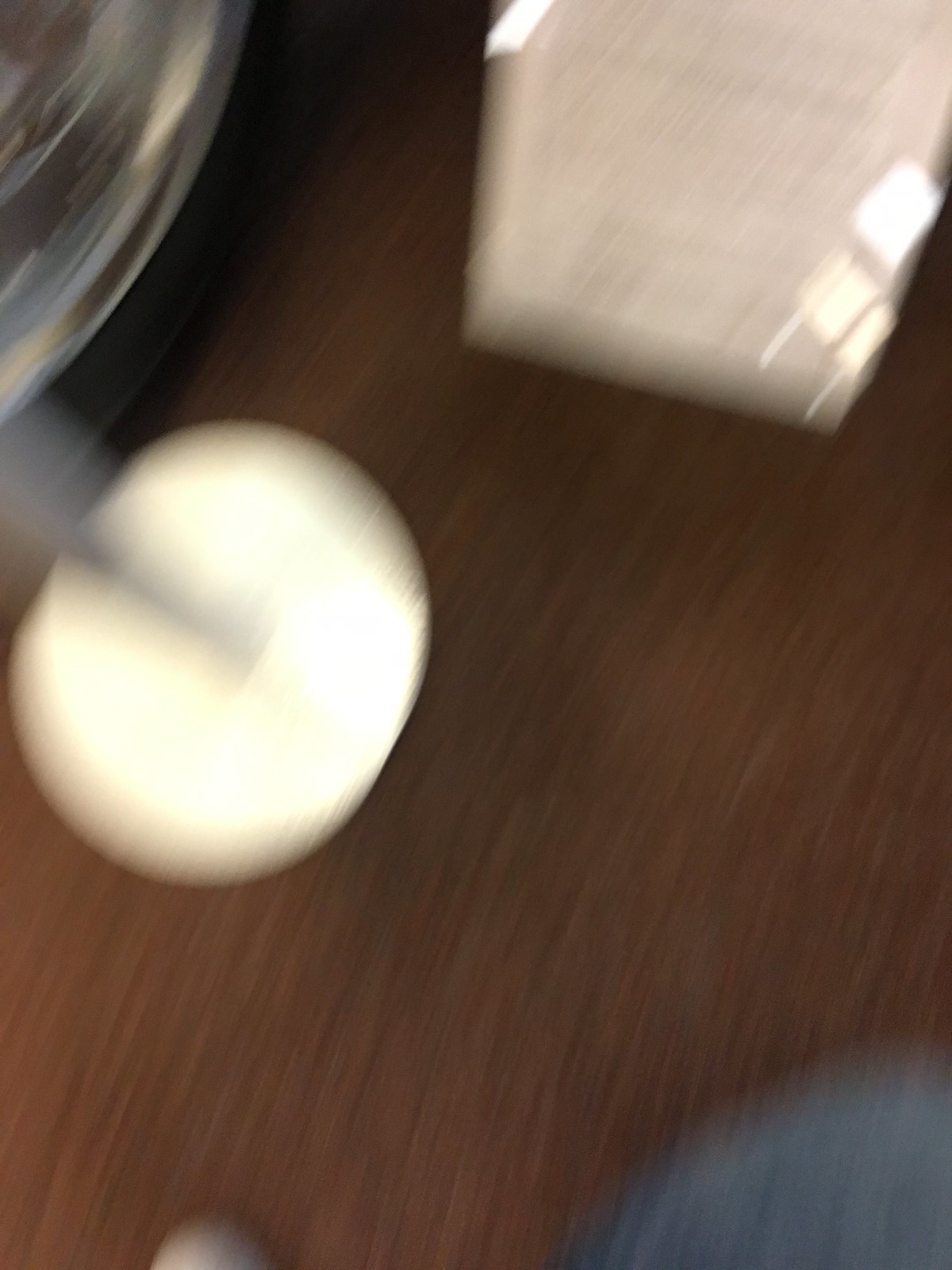The image is very blurry, making it challenging to discern specific details. The floor appears to be brown, possibly carpeted. Centrally, there's a glossy, circular object with a grey rod extending upwards. This could be the base of a Hawaiian glass piece. In the top right corner, there is a white, square object, and on the bottom left, an oblong-shaped white object can be seen. The left upper corner has another white object with gold and darker shades beneath it. The composition of the photo suggests it was taken accidentally, as there are no other objects, text, or distinct colors present.